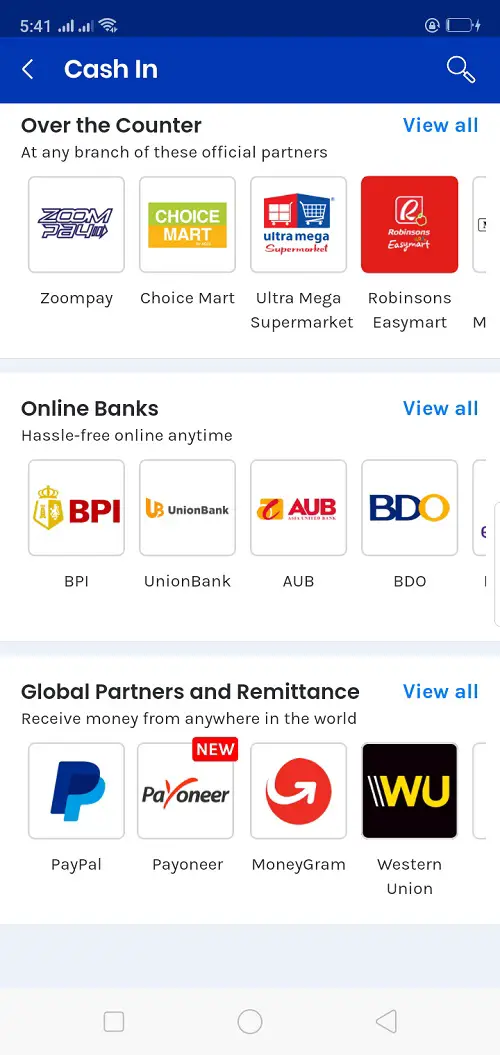The image portrays a user interface with a dark blue border at the top displaying the time (9:41) and an almost empty battery icon. Below, a lighter blue area contains a left-hand symbol and the text "Cash In," alongside a magnifying glass icon on the right. Beneath this, a white background section lists "Over the Counter" options with a blue "View All" hyperlink. It mentions availability at official partner branches, including Zoom Pay, Choice Mart, Ultra Mega Supermarket, and Robinson's Easy Mart, each represented with its respective logo and a box.

Further down, the section titled "Online Banks" features another blue "View All" hyperlink and promotes a "Hassle-Free Online Anytime" service. Four boxes display logos for BPI, Union Bank, AUB, and BDO. At the bottom, the image references "Global Partners and Remittance."